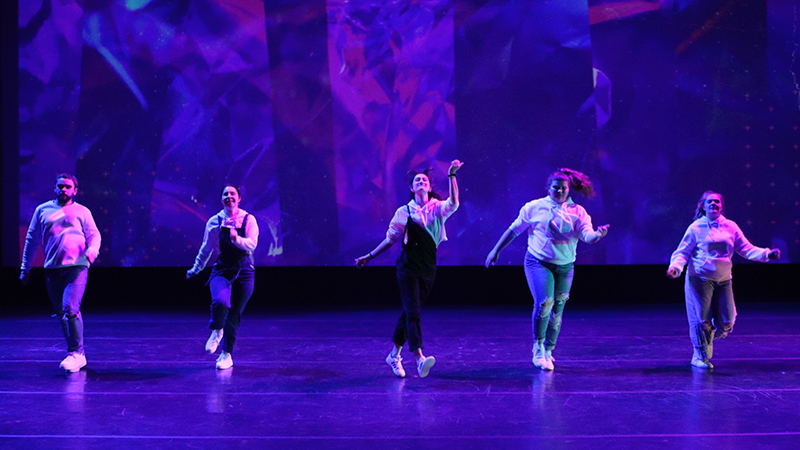This image is a landscape-oriented color photograph depicting five people dancing on a stage illuminated with deep blue and purple lighting. To the left side of the stage stands a heavyset man among four women. The man, situated on the far left, is smiling and appears to be part of a line dance. The woman second from the right also has a heavier build compared to the others. The center female, exuding joy, is dressed in dark overalls with only one strap fastened and has her fist in the air. She is looking up with a broad smile. The first girl to the man’s right sports overalls with both straps on, while the two women on the far right are in white sweatshirts, one with sleeves rolled up and the other with sleeves down. The group, collectively clad in various styles of jeans, is energetically lifting their arms and knees. They are positioned near the front of the stage, backed by a dynamic backdrop featuring multicolored abstract shapes in hues of purple, blue, and red, alongside darker horizontal panels. The setting conveys a vibrant and lively atmosphere, possibly capturing a moment from a live performance or a video freeze-frame.